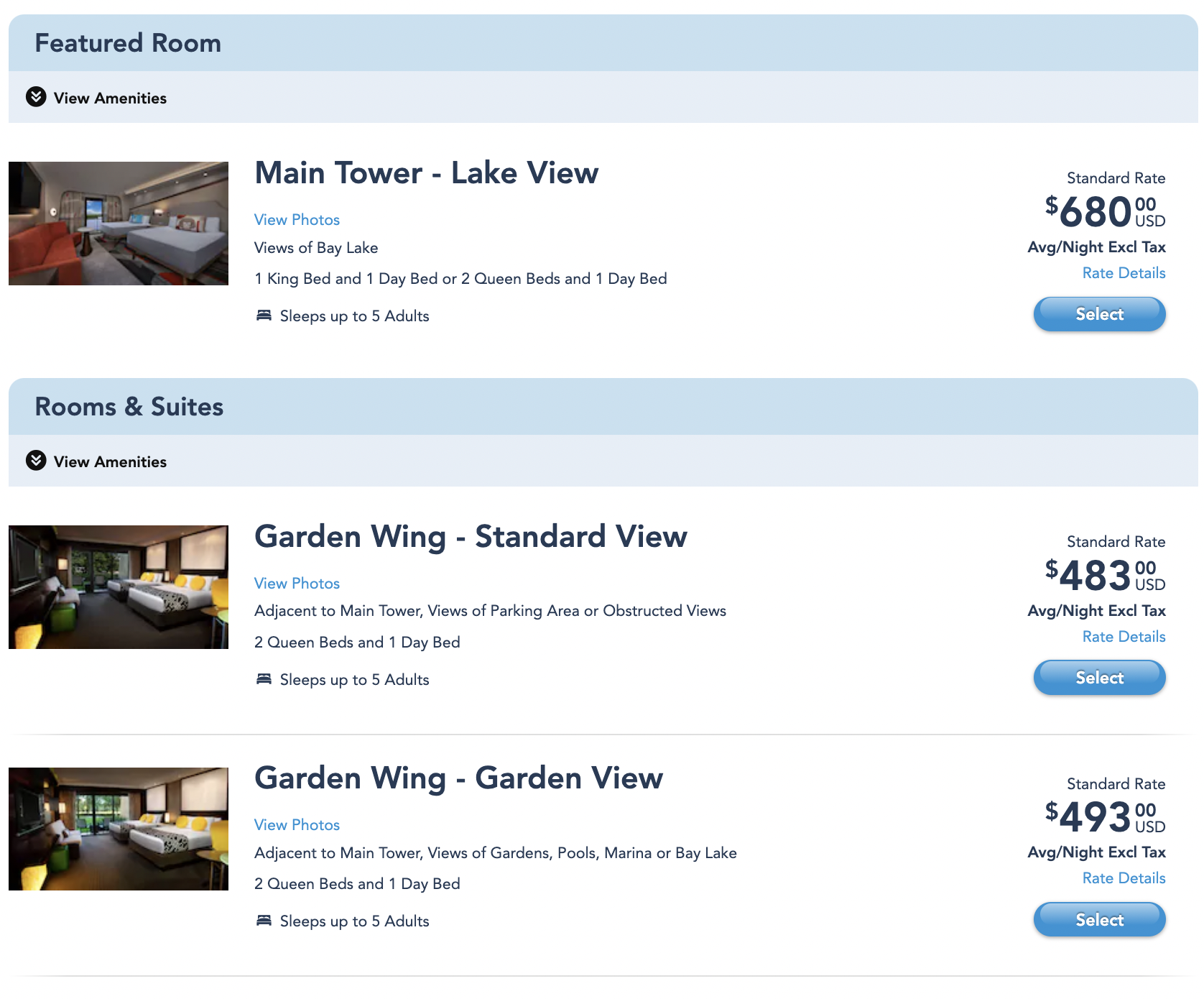This image is a detailed webpage from a hotel website, showcasing various room offerings and their amenities, pricing, and views. The page is titled "Featured Room" and offers a comprehensive menu of different room options available within the hotel, each accompanied by photos and descriptions.

**Main Tower Lake View**:
- **View**: Bay Lake
- **Bed Options**: One king bed and one day bed, or two queen beds and one day bed
- **Capacity**: Sleeps up to five adults
- **Pricing**: Standard rate $680 per night (average, excluding taxes)

**Garden Wing, Standard View**:
- **View**: Adjacent to Main Tower; views of parking area or obstructed views
- **Bed Options**: Two queen beds and one day bed
- **Capacity**: Sleeps up to five adults
- **Pricing**: Standard rate $483 per night (average, excluding taxes)

**Garden Wing, Garden View**:
- **View**: Adjacent to Main Tower; views of garden pools, Marina, or Bay Lake
- **Bed Options**: Two queen beds or one day bed
- **Pricing**: Standard rate $493 per night (average, excluding taxes)

Each room listing features an option to view more photos and further rate details. This structured layout allows potential guests to easily compare and select the room that best fits their preferences and budget.